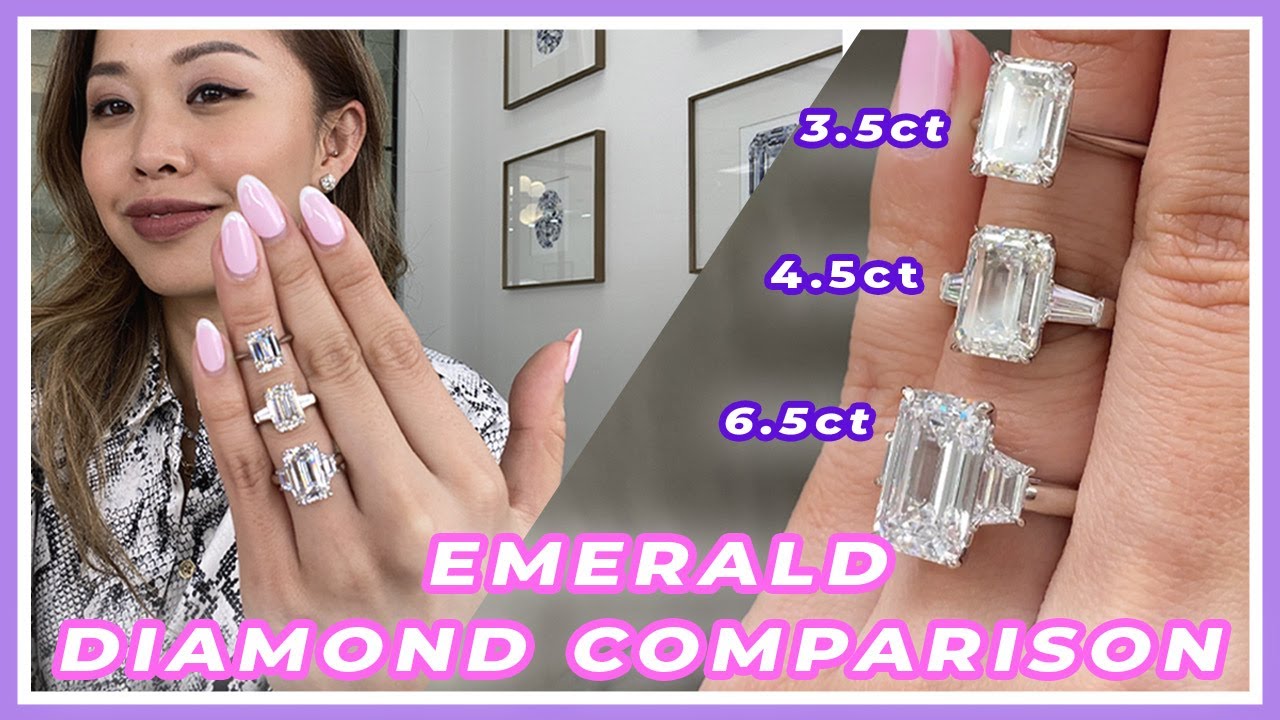This horizontal advertisement for Emerald Diamond Comparison, outlined in purple and white, features an Asian woman with long, brown hair and dark, berry-red lips. She is dressed in a stylish black and white snakeskin print top. On the left side of the image, she smiles while holding up her left hand, displaying three diamond rings on her well-manicured ring finger, which features light pink nails with white French tips. The white-walled background with hanging pictures adds to the composition.

The image is split diagonally, transitioning to a close-up of her hand on the right side. This close-up highlights the three rings with rectangular diamonds, each set in silver bands. The top ring is labeled "3.5 CT" in purple and white text, the middle ring is labeled "4.5 CT," and the bottom and largest ring is labeled "6.5 CT." At the bottom of the image, in eye-catching white letters outlined in bright pink, the text reads "Emerald Diamond Comparison."